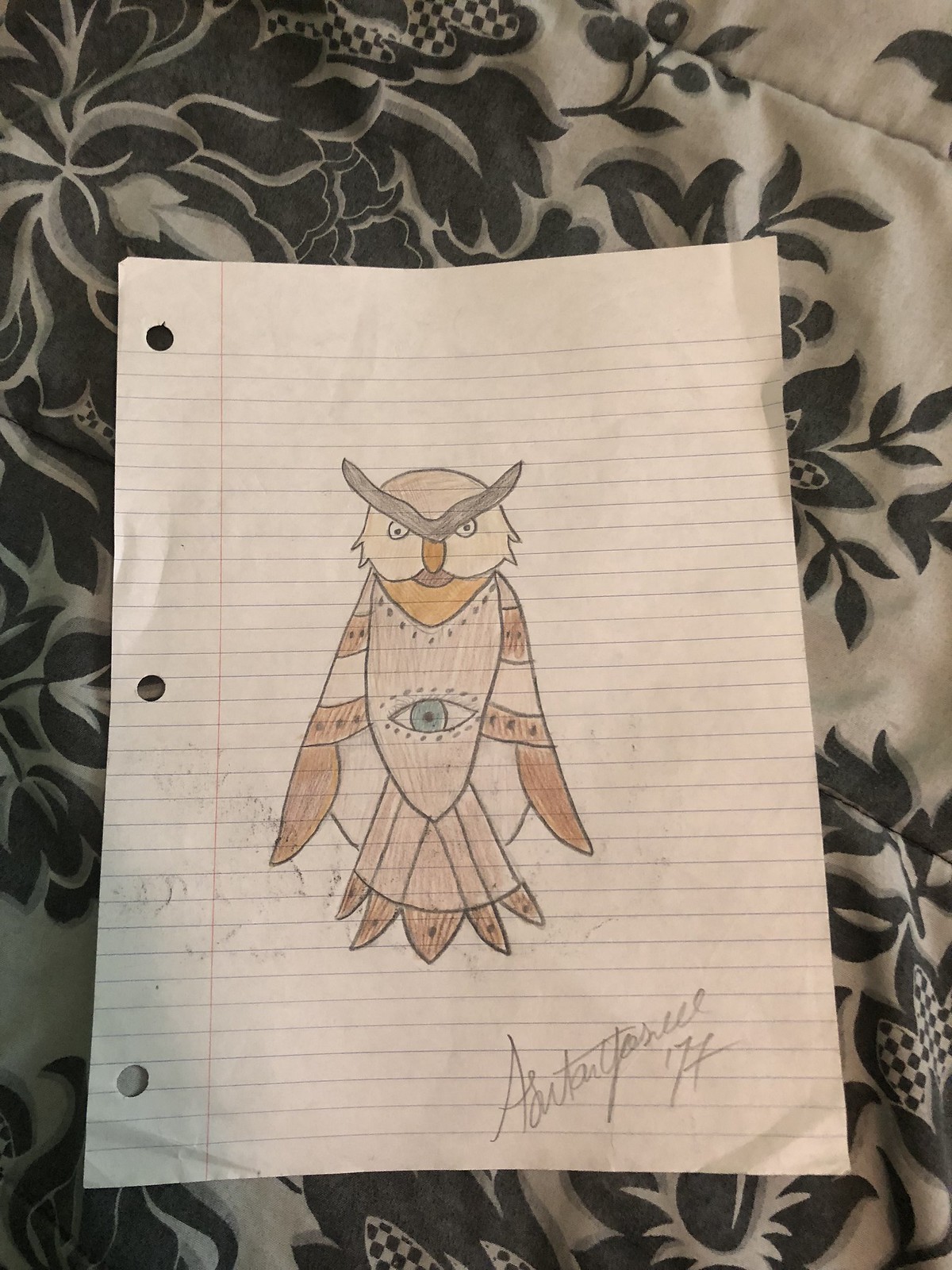The image depicts a detailed drawing on a piece of lined paper, which is laid out on a soft surface featuring a black and white floral pattern, probably a blanket or comforter. The paper has three punched holes along its left margin, indicating it could be placed in a binder, and horizontal blue lines with a vertical red line near the holes. The drawing itself is of a mythical, fantasy-like brown owl facing forward directly at the viewer. This owl has a unique set of thick, connected brown eyebrows resembling a unibrow, an orange beak, and patterned feathers. The feathers on its wings are striped with alternating dark brown and white segments, and black dots are aligned horizontally on the brown stripes. Distinctively, there is a light blue eye in the center of its torso, surrounded by dots. The artist’s signature is visible at the bottom right of the drawing, although it is difficult to decipher clearly.